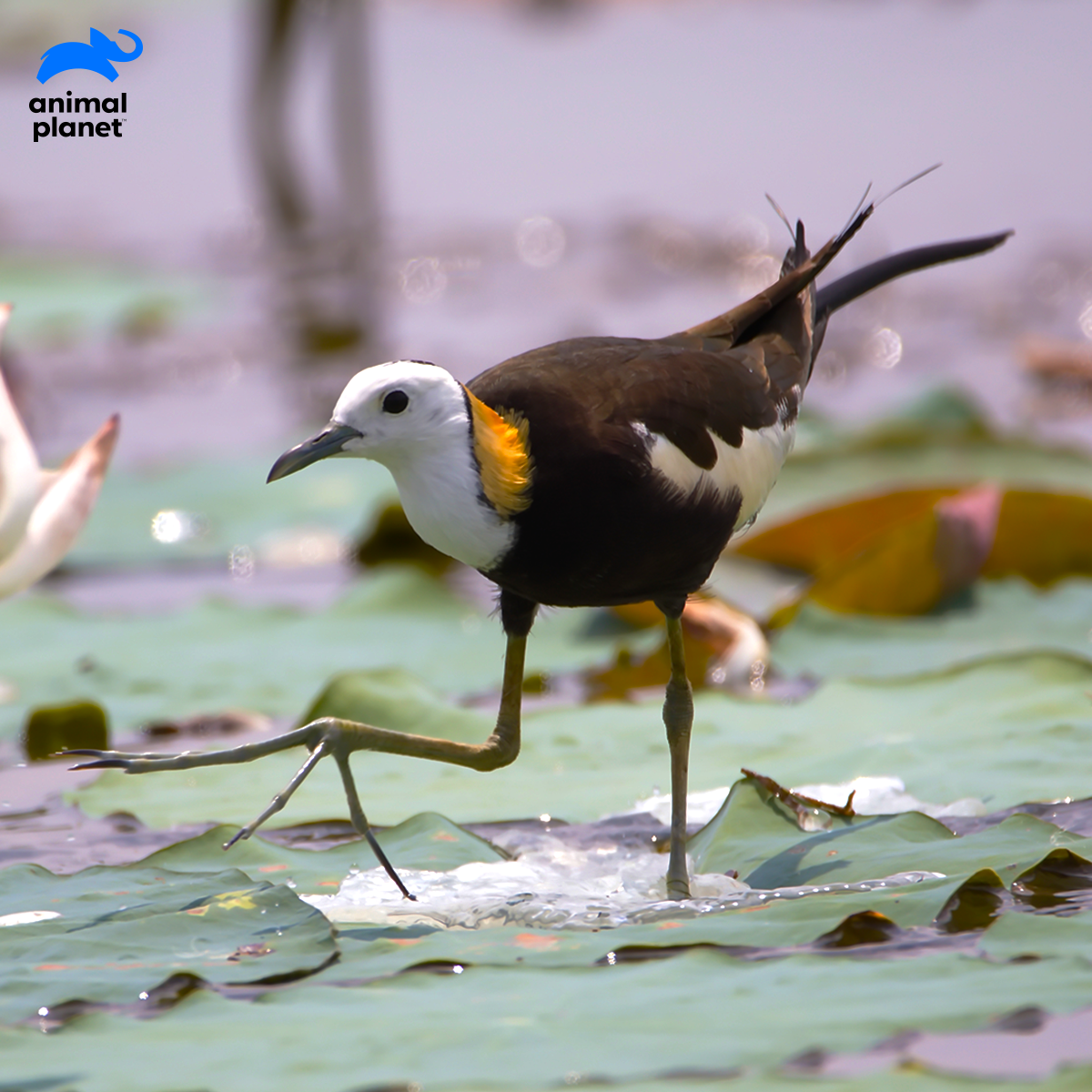This professional photo features a peculiar bird standing atop lily pads in a shallow pond, with water only reaching its ankles. The bird, reminiscent of a cross between a seagull and a dove, exhibits strikingly disproportionate features. Its elongated yellow legs support massive, raptor-like feet with long, gray toes lacking webbing. The body is predominantly dark brown with white markings on the underside, presenting an elegant contrast to its colorful head. The bird’s head is predominantly white with a pronounced grayish, medium-sized, pointy beak, and a distinctive, bright yellow patch adorns the nape, transitioning to a reddish hue. Its right eye, keenly directed toward the camera, enhances the bird's intriguing appearance amidst the serene water lilies, underscoring its unique and captivating nature. The top left corner of the photo also includes a blue elephant logo and the "Animal Planet" branding, indicating its professional origin.